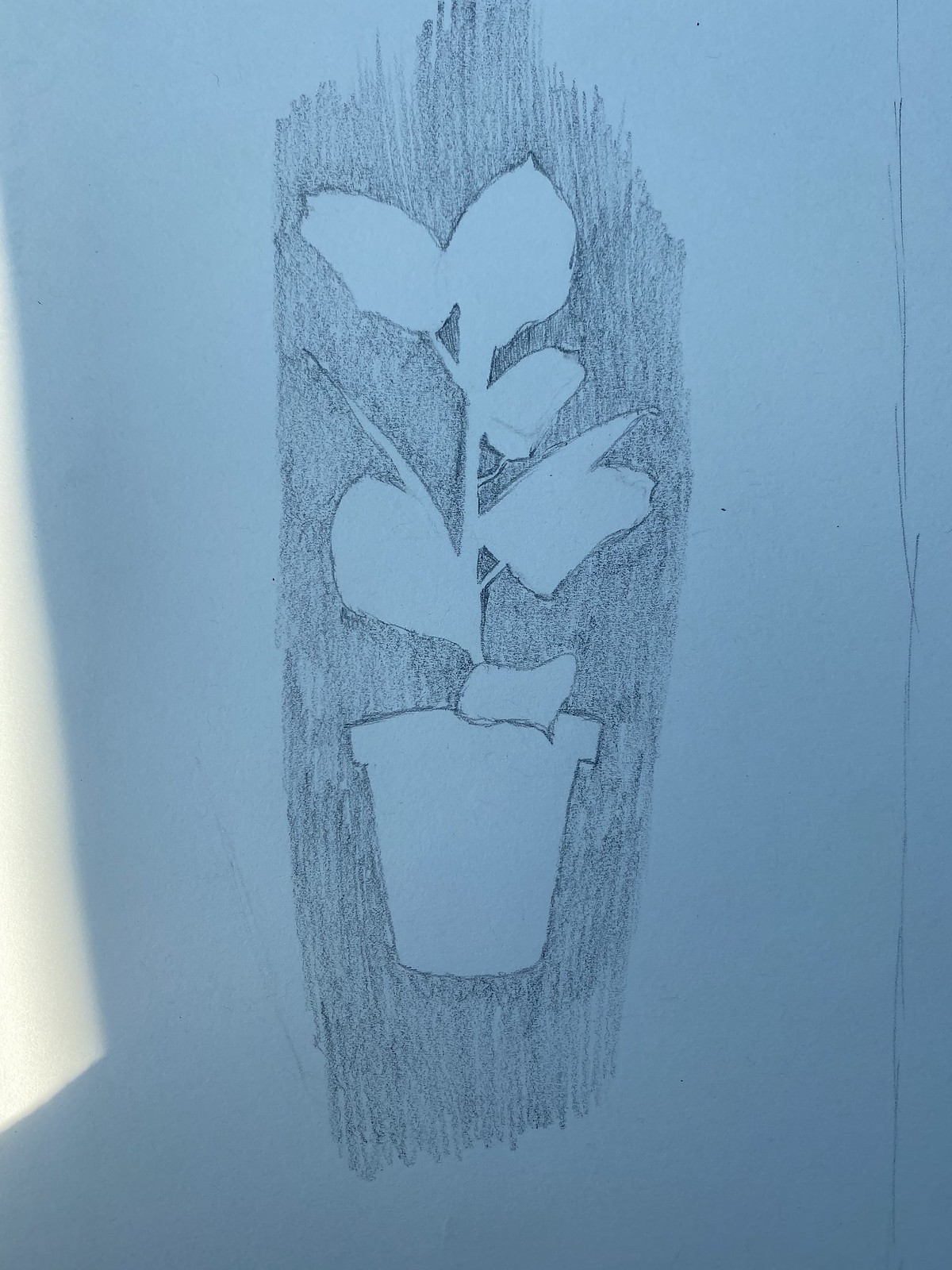This is a color photograph of an intricately detailed drawing that occupies nearly the entire frame. The drawing is rendered on stunning sky blue paper, which features subtle gradations, with the upper portion of the paper appearing slightly lighter than the deeper blue at the bottom. The artwork seems to be created using pencil or charcoal, characterized by delicate etching and extensive shading.

The focal point of the drawing is an elegantly outlined house plant. It is placed in a traditional clay pot with a classic rim, meticulously detailed to highlight its texture. The house plant itself is tall with impressively large leaves, each leaf boasting finely executed shading to accentuate its form and depth. This exquisitely rendered composition, though simple, exudes a captivating beauty.